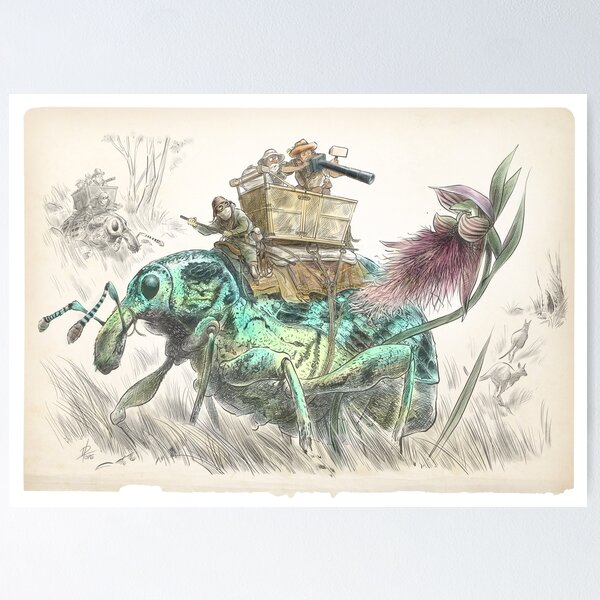This surreal colored pencil drawing showcases an enormous beetle, akin to the size of an elephant, with a teal hue that transitions to a light, lime green shade on its stomach. The beetle also features a distinct yellow belly and a prominent eye, and it appears to be facing left. Towering over the scene, the beetle's back is adorned with a basket-like carriage, reminiscent of those used on elephants for safaris. Inside the carriage sit two men, one equipped with a camera with an exaggeratedly long telescoping lens, possibly aiming to capture an image of a large, striking purple flower the beetle seems to be interacting with. Next to the photographer is another man, possibly an explorer, characterized by a bushy white beard and an explorer's hat. Controlling the beetle, a third man rides on a saddle positioned in front of the basket. The background is a light beige-pink canvas with charcoal details, giving a pencil-sketched ambiance to the overall scene, including grassy patches that almost resemble hair. Additional details include a pair of pencil-sketched kangaroos at the bottom right and another similar, albeit black and white, beetle in the back left corner of the image. The overall composition suggests a whimsical safari adventure set in a world where giant beetles serve as the mode of transport.